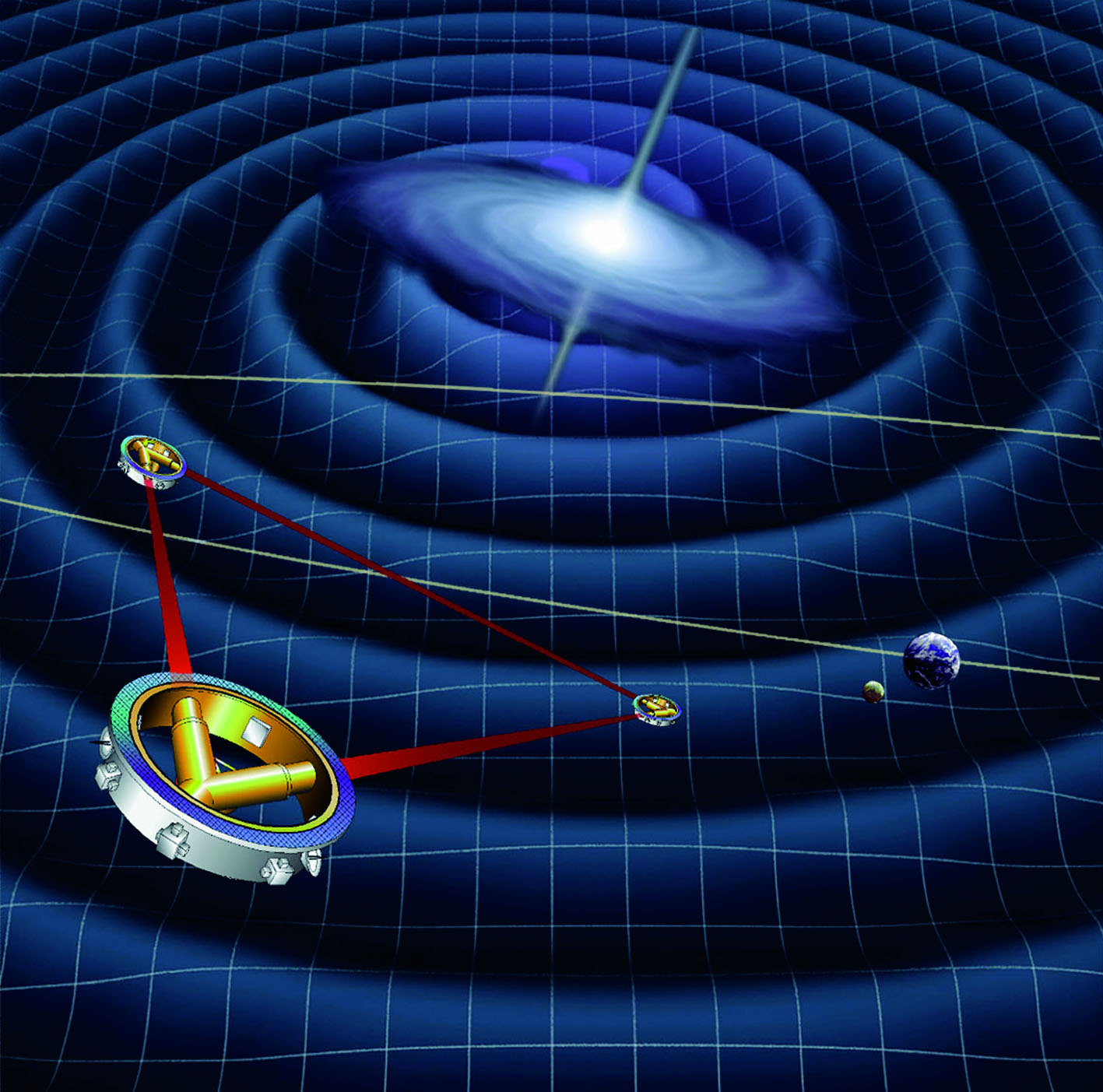This image appears to be a complex, computer-generated graphic with a distinctly digital aesthetic, reminiscent of early internet or electronic graphics, characterized by a gritty, grid-like texture in the background. The backdrop features a main element that captivates the viewer: a swirling blue spiral resembling a galaxy, centered by a radiant white light. Radiating from this central point are white lines, adding a sense of dynamic motion.

In the upper section of the image, this spiral form assumes a whirling, dervish-like appearance, accented by two protruding spikes. In the middle-left section, there’s a small depiction of Earth accompanied by its Moon, interconnected by a yellow line, suggesting an orbital path within this fantastical cosmos.

Dominating the middle and right portions of the image is an intricate triangular structure made up of metallic-looking silver and gold pieces, connected at each vertex by red triangular signs. This geometric formation appears to have mechanical elements, including what might be interpreted as pistons or lasers within its design. The entire composition evokes a futuristic, almost otherworldly scene where Earth's traditional imagery mingles with advanced, possibly extraterrestrial constructs amid a rippling cosmic background.